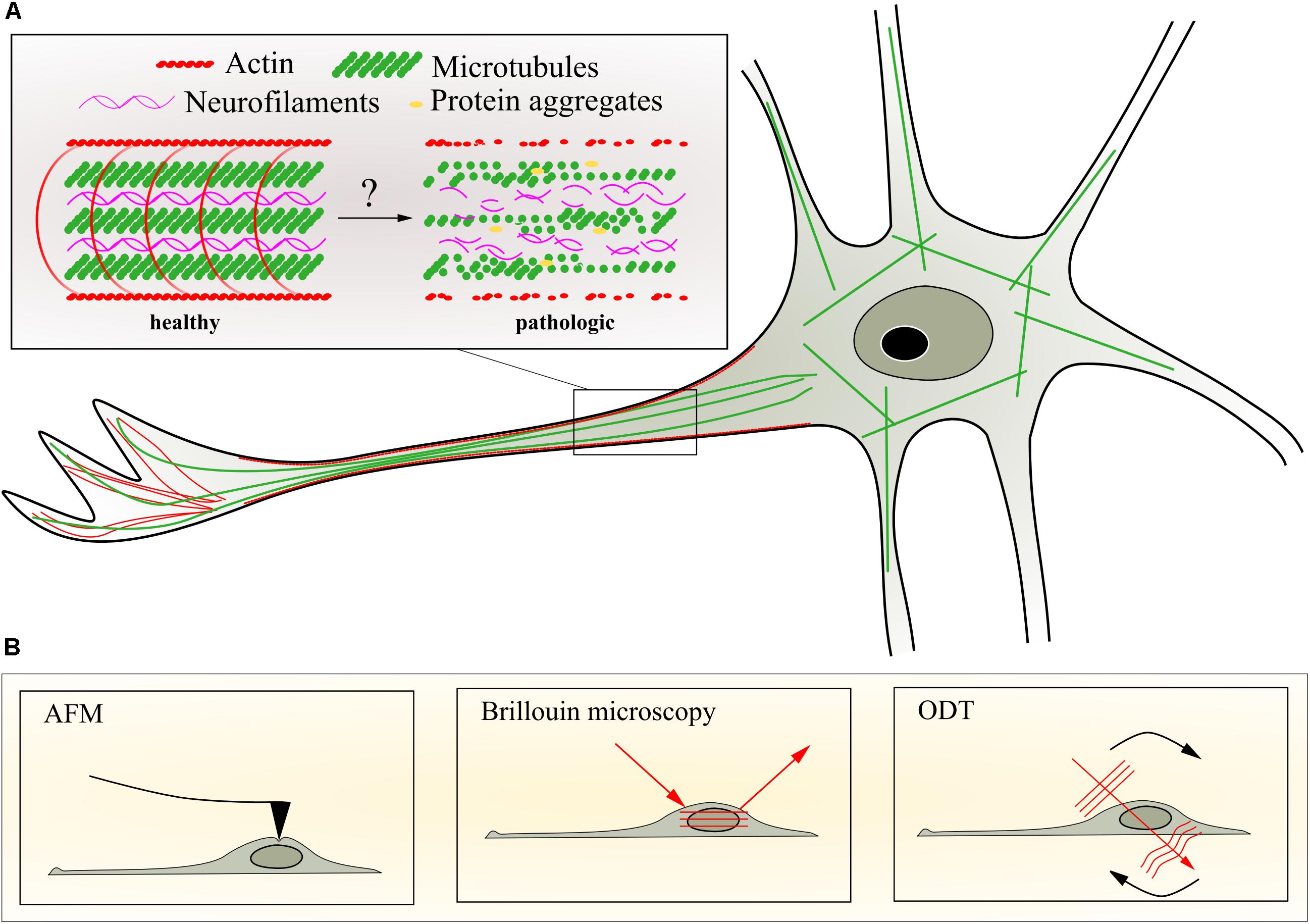This detailed scientific diagram appears to be from a textbook, illustrating aspects of cellular anatomy. The diagram is divided into two main sections, labeled A and B. 

### Section A:
In the top-left corner, labeled as A, there's a white box with a black outline containing various terms: "Actin, Neurofilaments, Microtubules, Protein Aggregates." This section contrasts healthy and pathologic conditions. On the left side, indicating "healthy," the figures include little red dots at the top, green slashes across three rows, and wavy purple lines in between, with green dots on the right side. In contrast, the right side, indicating "pathologic," displays similar shapes rearranged differently, highlighted by an arrow with a question mark pointing to them.

### Section B:
The bottom section, labeled as B, features three smaller boxes named AFM, Brillouin Microscopy, and ODT. Each of these boxes contains stylized scientific sketches with arrows indicating various directions, reflective of cellular pathways and processes. The illustrations in B demonstrate different aspects and techniques for examining the structures detailed in section A.

### Central Illustration:
The middle of the diagram, not enclosed by a box, depicts a large, grayish-green, oval-shaped structure resembling a nerve cell or ganglion. This central figure, which almost looks like it has an eyeball in the middle, is dynamic with straight green lines forming a trapezoid around it. This figure ties together the structural elements from A and B, showing the interconnectedness of healthy and pathological cells, as well as representing different microscopy techniques.

Overall, the illustration uses colors like red, green, and purple to differentiate various components, aiming to provide an educational comparison between healthy and diseased cellular structures and the methodologies used to study them.